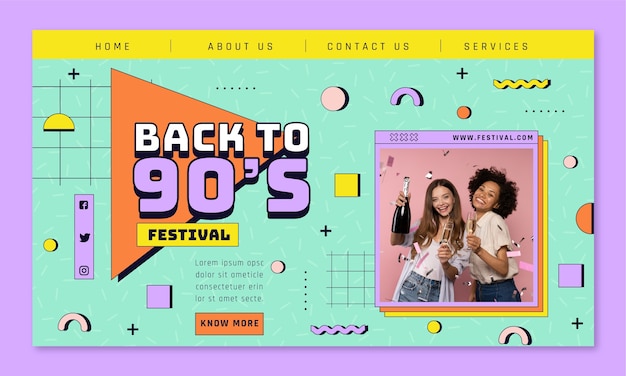This detailed, descriptive caption incorporates the shared and repeated elements of the image:

The advertisement for the Back to 90s Festival is designed in a nostalgic early 90s website style, featuring a pale purple border with a yellow top bar. The website-inspired layout is divided into four sections by vertical black lines: Home, About Us, Contact Us, and Services. The festival name is prominently displayed in three distinct fonts: "Back 2" in white block letters with a drop shadow, "90s" in large purple block letters with a drop shadow, and "Festival" in bold black text inside a yellow rectangle. Below the festival name is placeholder text reading "Lorem Ipsum," followed by an orange rectangle labeled "KNOW More." On the left side, a purple rectangle houses Facebook, Twitter, and Instagram logos. The right side features a photograph of two young ladies holding a wine or champagne bottle and toasting with champagne glasses against a pink background. The upper border includes "www.festival.com" on the right and three X's on the left. Scattered around the image are colorful shapes such as arches, squiggles, circles, and semicircles in pink, purple, yellow, and orange, adding to the retro vibe. The overall color scheme includes pale purple, dark yellow, and mint green, enhancing the nostalgic feel of the advertisement.